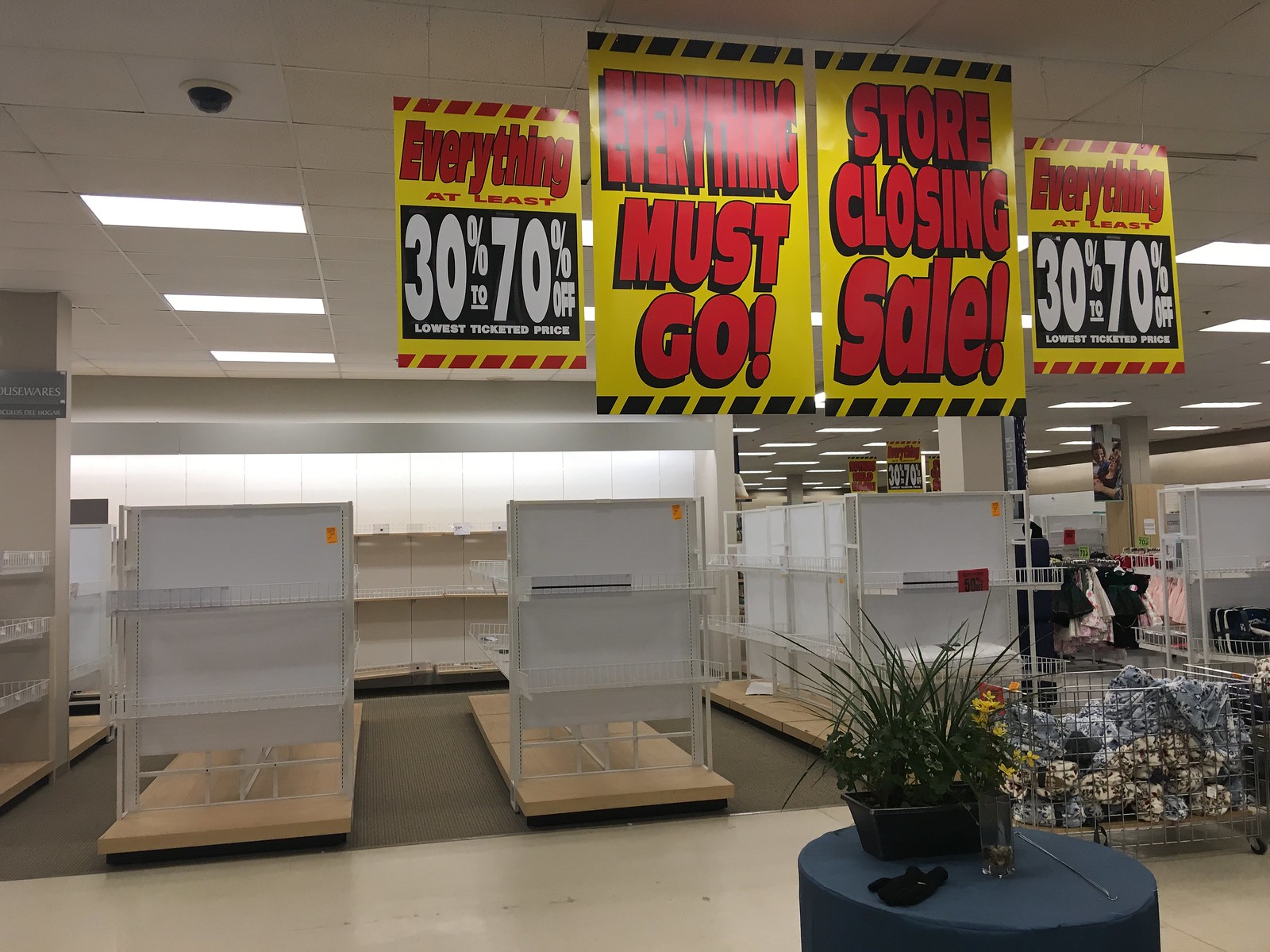A somber scene of a clearance sale in a clothing store. The image reveals numerous empty sales racks and shelves, indicating a significant reduction in inventory. In the foreground, there is a blue round table adorned with flower arrangements, adding a touch of contrast to the otherwise desolate surroundings. Nearby, a cage-like display holds some items still on sale. Overhead, bold yellow and red signs announce, "Everything Must Go," with discounts ranging from 30-70% off the lowest ticketed prices. The sale signs, featuring warning dots along the edges, vary in detail: smaller signs have red dots, while the larger signs are marked with black dots. The racks and displays are arranged on a carpeted floor, with no visible clear pathways for walking through the store.